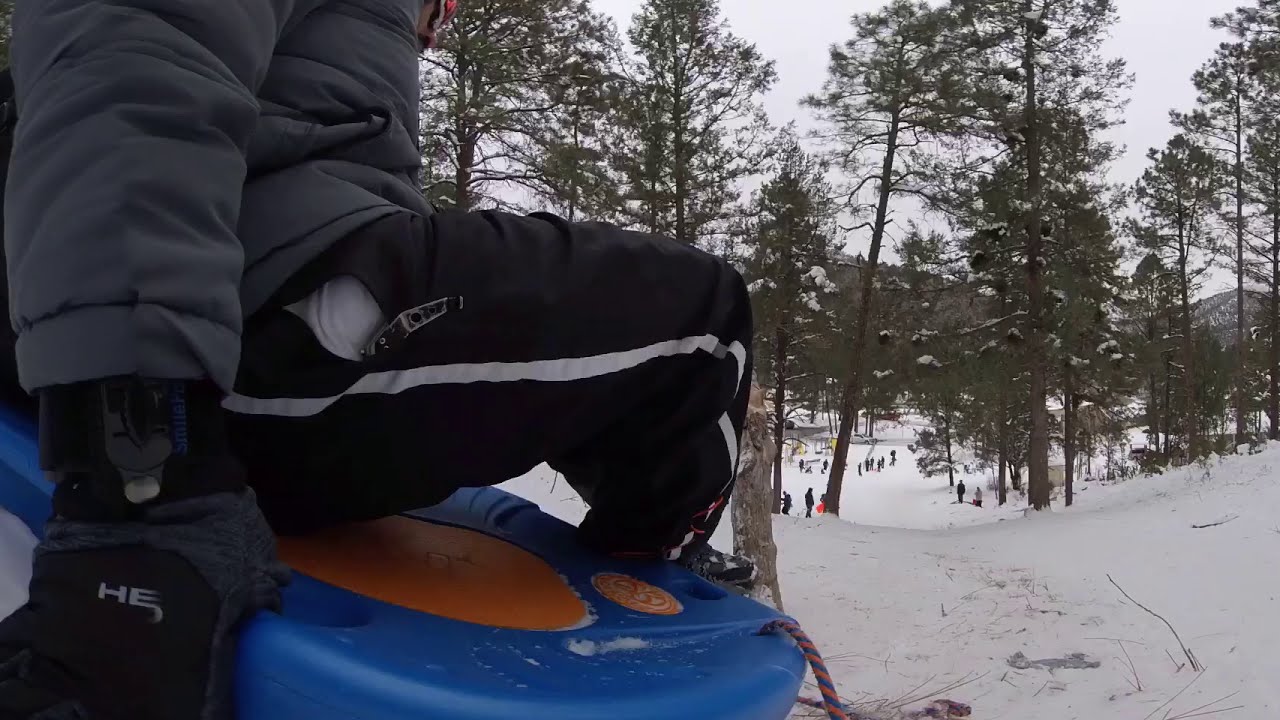In this wintry scene, set against a snowy terrain with scattered evergreen trees and distant mountains, the focus is on an individual sledding down a snow-covered hill. The photo captures the person from behind as they navigate a well-trodden pathway between the trees. The sledder is seated on a blue and orange sled, gripping its blue and orange rope. Dressed warmly for the cold weather, they sport a gray snow jacket, light black pants with white pinstripes down the sides, black gloves emblazoned with the letters "HE," and an orange cap with sunglasses shielding their eyes. The sled appears to be tethered by a rope that snakes its way down to the busy flat area at the hill's base, where numerous other people are gathered, enjoying the snowy outdoors.